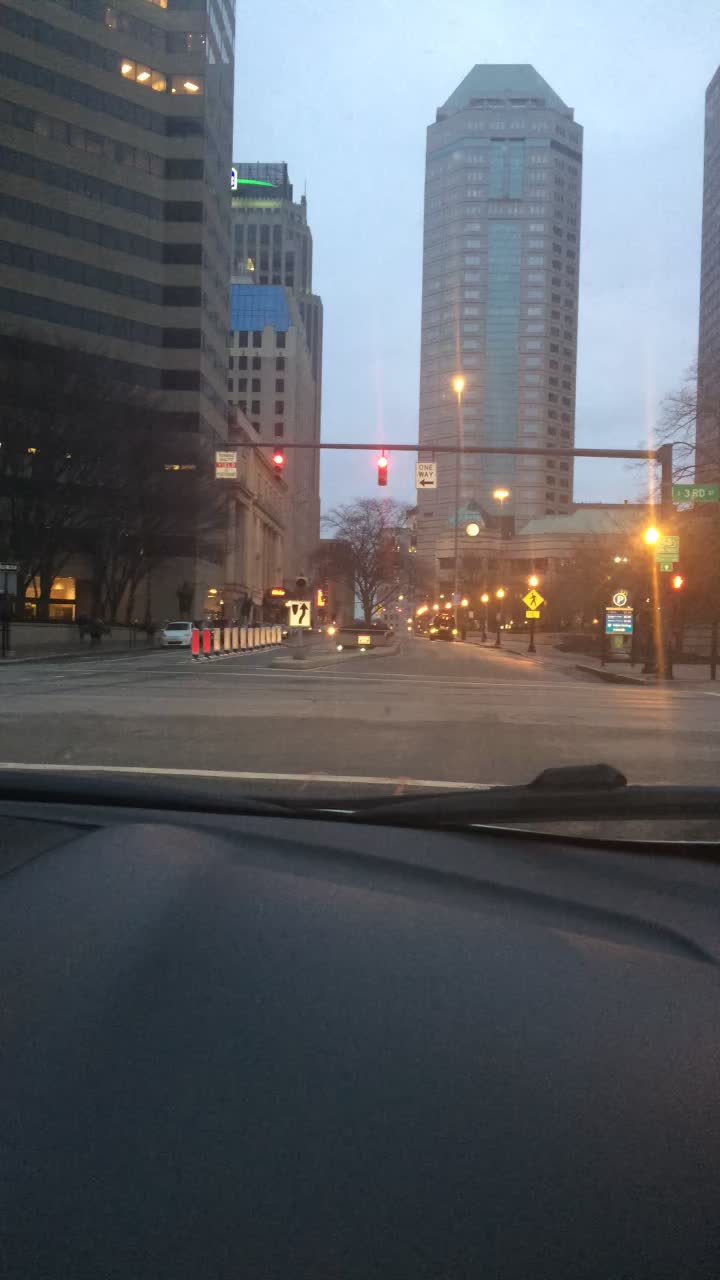The image captures a street scene from the perspective of a vehicle's driver or passenger. Ahead of the vehicle, a stop sign and a red traffic light are visible at an intersection, with a "One Way" sign indicating leftward direction. The background features towering office buildings typical of a downtown area, characterized by large facades with numerous windows. Several offices within the high-rises are illuminated, suggesting activity inside. Streetlights line the sidewalk, contributing to the urban aesthetic of the bustling cityscape.